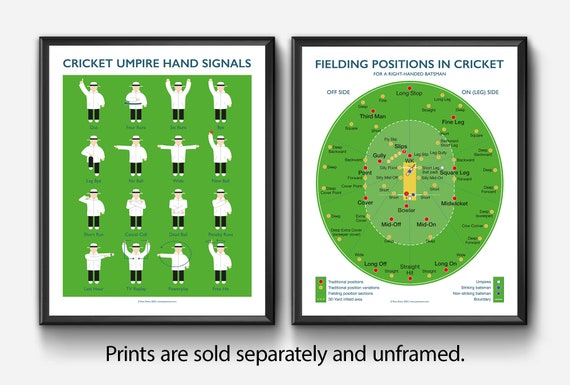This image features two side-by-side cricket-themed posters in thin black frames against a white wall, showcasing detailed cricket umpire hand signals and fielding positions. The left poster, titled "Cricket Umpire Hand Signals," displays a Caucasian male umpire wearing a white hat with a brim, a matching white jacket, black pants, and white shoes. Arranged in a 4x4 grid, there are 16 illustrations of him demonstrating various hand signals, all set against a predominantly green background. The right poster, titled "Fielding Positions in Cricket," features a large green oval that represents a cricket field. This oval is populated with yellow and red dots, each labeled with small black text to indicate specific fielding positions. Both posters have dark blue text headers and contain legends for further clarification. At the bottom of the image, there is a text stating that the prints are sold separately and unframed, suggesting a poster sale or advertisement.